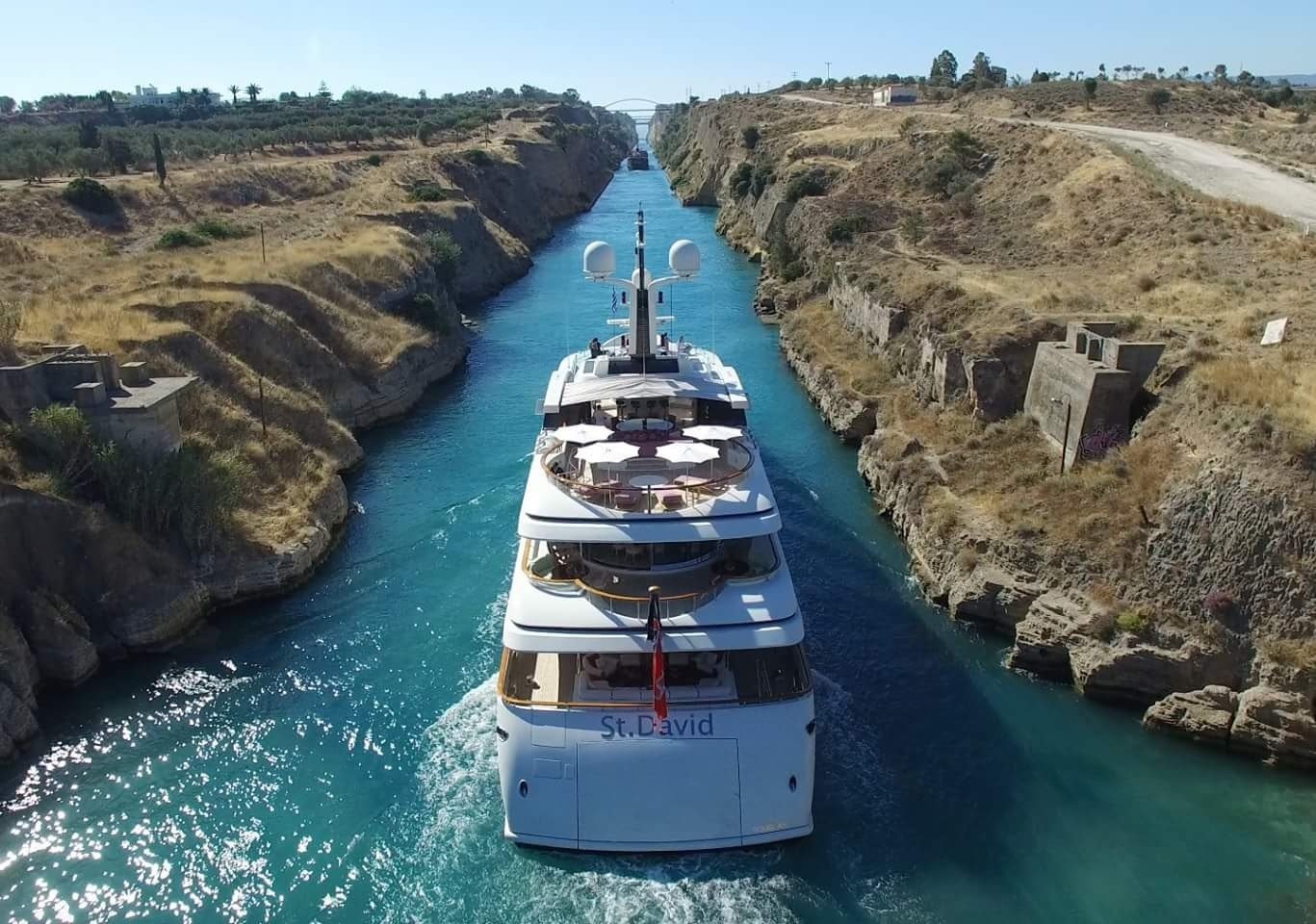This is a daytime aerial photograph, likely taken by a drone, capturing a white ferry named "St. David" navigating through a narrow, rocky canal. The waterway, surrounded by high rocky ledges topped with flat grassy land, appears to be a vivid aqua blue. The ferry, with at least three decks and an antenna equipped with radar or sonar equipment on the top forward deck, shows signs of propulsion as water churns in its wake. The stern of the ship is in the foreground, with the bow facing away from the camera. A second ship is visible in the far corner of the image, near a bridge. Flanking the waterway are steep, rocky hills and sparse vegetation, with a paved roadway following the canal's path on the upper right side. The backdrop features a flat horizon lined with tall trees and a bright blue sky. There are people visible on the ferry, enjoying the sunny day.